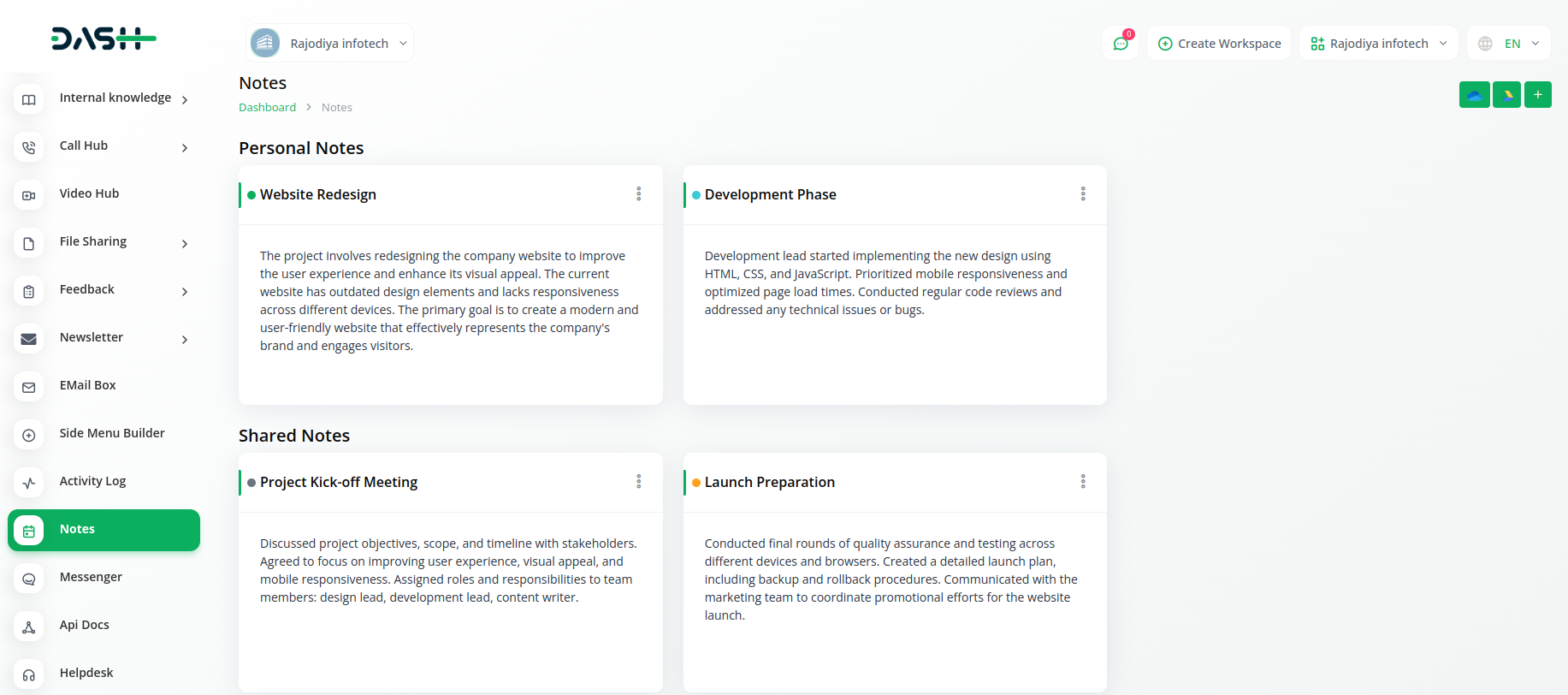This screenshot captures a user interface from an internal platform. The word "Dash" is prominently displayed in the upper left-hand corner. A vertical menu on the left side of the page includes several navigation options: Internal Knowledge, Call Hub, Video Hub, File Sharing, Feedback, Newsletter, Email Box, Side Menu Builder, Activity Log, Notes, Messenger, API Docs, and Help Desk. Currently, the "Notes" option is highlighted with a green rectangular box.

On the main section of the screen, the "Notes" interface specifically pertains to Rajadia Infotech. The personal notes section offers different categories, such as notes for website redesign and development phase. In the shared notes section, two key notes are listed: "Project Kickoff Meeting" and "Launch Preparation." The "Launch Preparation" note details critical activities undertaken, including the final rounds of quality assurance and testing across various devices and browsers, the creation of a comprehensive launch plan that incorporates backup and rollback procedures, and communication with the marketing team to synchronize promotional efforts for the impending website launch.